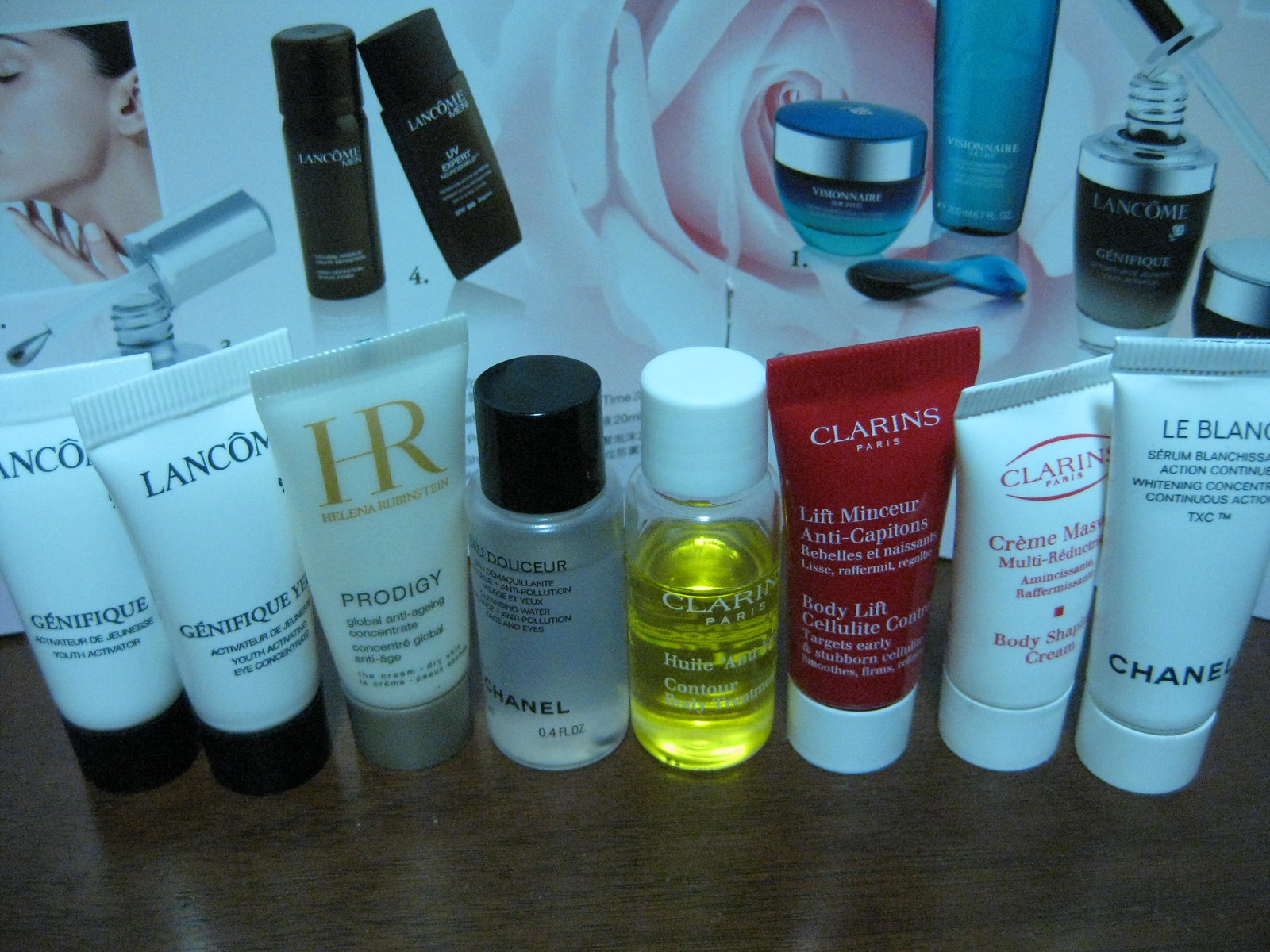This photograph captures a meticulously arranged assortment of beauty products on a polished brown table. On the far right, there's a sleek white bottle with black writing labeled "LE BLANC" by Chanel. Next to it is a white tube of Clarins body cream. Beside the Clarins product, a striking red tube with a white lid stands out. Adjacent to the red tube is a clear tube containing a yellow liquid, capped with a white lid. Following that, there is another clear tube, this one with a black lid and black writing. Continuing from there, a white tube with a gray cap is visible. Completing the lineup are two identical white tubes each featuring black writing and a black lid. In the background, the wall is adorned with posters showcasing flowers and an array of face creams and other skincare products in jars and tubes, adding context to the beauty theme of the image.